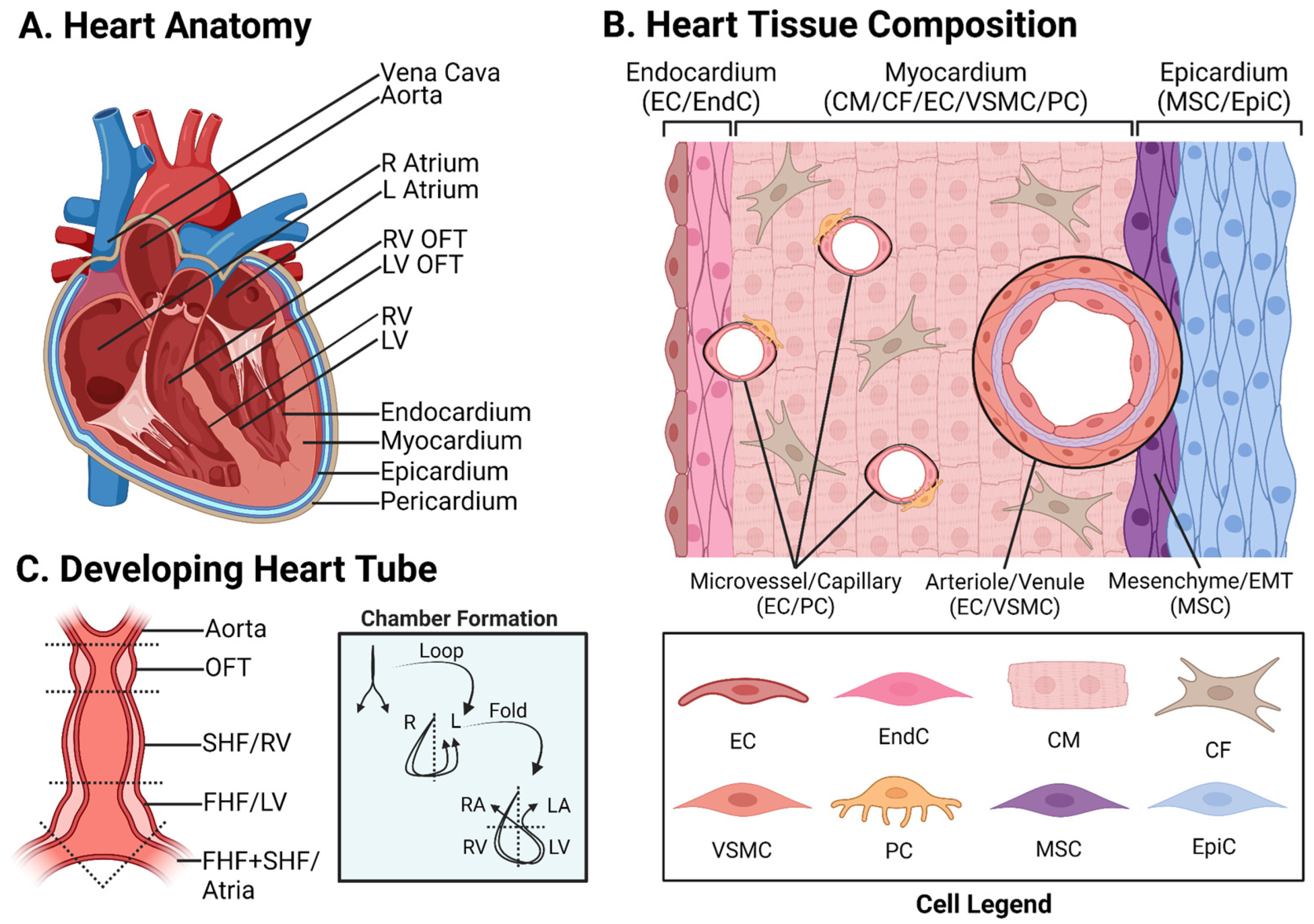The image depicts a detailed anatomical and developmental diagram of the human heart, labeled with three main sections: Heart Anatomy (A), Heart Tissue Composition (B), and Developing Heart Tube (C).

Section A, Heart Anatomy, displays a schematic of the heart's structure highlighting essential components such as the vena cava, aorta, and the right (R) and left (L) atriums. The diagram is color-coded, showcasing red arteries and blue veins. It also delineates the heart layers: endocardium, myocardium, epicardium, and pericardium, with arrows indicating their locations.

Section B, Heart Tissue Composition, offers a close-up, colored cross-section of the heart tissues. It vividly demonstrates the distinct layers—endocardium, myocardium, and epicardium—using various colors like blue, pink, and orangish hues. This part also includes a cell legend representing different cell types (EC, NC, CM, CF, VS, MC, PC, MSC, and Epi C), which are illustrated with diverse shapes and colors to clarify cellular composition.

Section C, Developing Heart Tube, illustrates the progression of the heart tube's development, often resembling a tubular structure. Labels identify various stages and components such as the aorta, OFT (Outflow Tract), SHF (Second Heart Field), RV (Right Ventricle), and FHF (First Heart Field). The diagram shows how these parts evolve and interact, exhibiting complex developmental stages within a single schematic.

Overall, the diagram serves as an educational tool, detailed with multicolored visual aids and black text annotations to illustrate the anatomy, tissue composition, and development of the heart seamlessly.